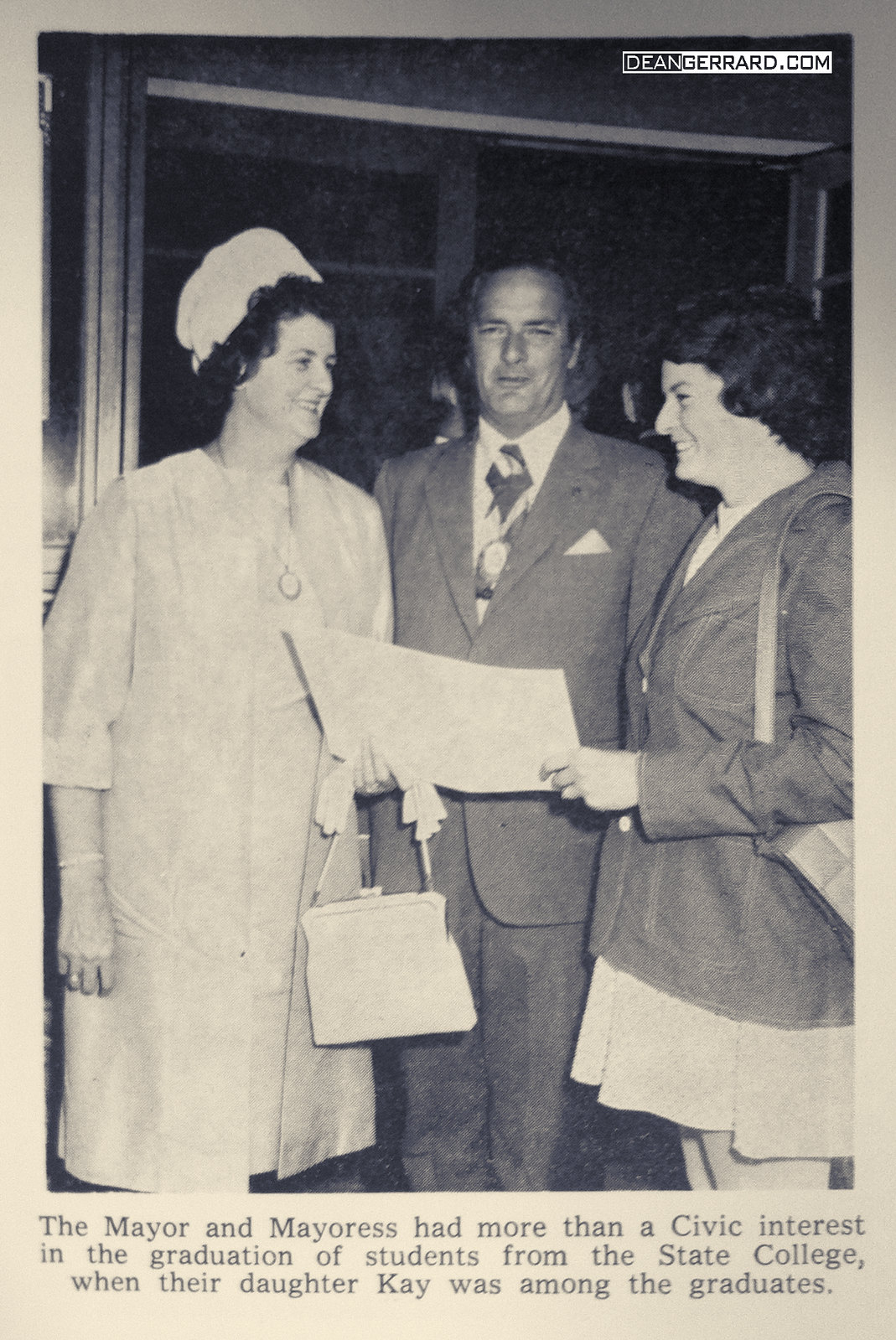This black-and-white newspaper clipping from the 1950s features three individuals: a man in the center and two women on either side of him, all in their forties. The man, wearing a suit and patterned tie, stands between the women, who appear to be showing him a certificate they're jointly holding across him. The woman on the left is elegantly dressed in a white dress with a matching box hat and short curled hair, accessorized with a large pendant necklace, white purse, and gloves. The woman on the right, presumably their daughter, Kay, has bobbed, wavy dark hair and is dressed in a darker blazer with either a dress or skirt, also holding a purse. Both women are looking at each other with smiles, while the man gazes straight ahead at the camera. The caption beneath the photo reads: "The mayor and mayoress had more than a civic interest in the graduation of students from State College when their daughter Kay was among the graduates," indicating the familial connection among the trio.